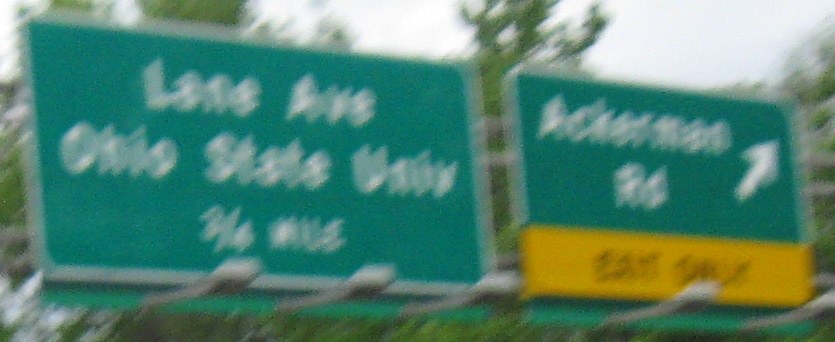This image depicts a blurred photograph of two freeway signs, presumably taken from a moving vehicle. Both signs are green with white borders and white text, mounted on a high metal pole for visibility to passing drivers. 

The left sign is a slightly longer rectangle and, despite the blur, you can decipher "Lane Avenue" on the first line, followed by "Ohio State University" on the second, and "3/4 mile" on the third, although the word "mile" is not entirely clear. 

To the right, a shorter rectangular sign reads "Ackerman Rd" with a diagonal arrow pointing to the top right. At the bottom of this sign, there is a yellow bar with black text indicating "exit only," though it is hard to discern due to the blur. 

In the background, it is daytime with visible green trees, though the sky appears gray and overcast. The image fills the entire frame, emphasizing the prominence of these freeway directions against the roadside backdrop.